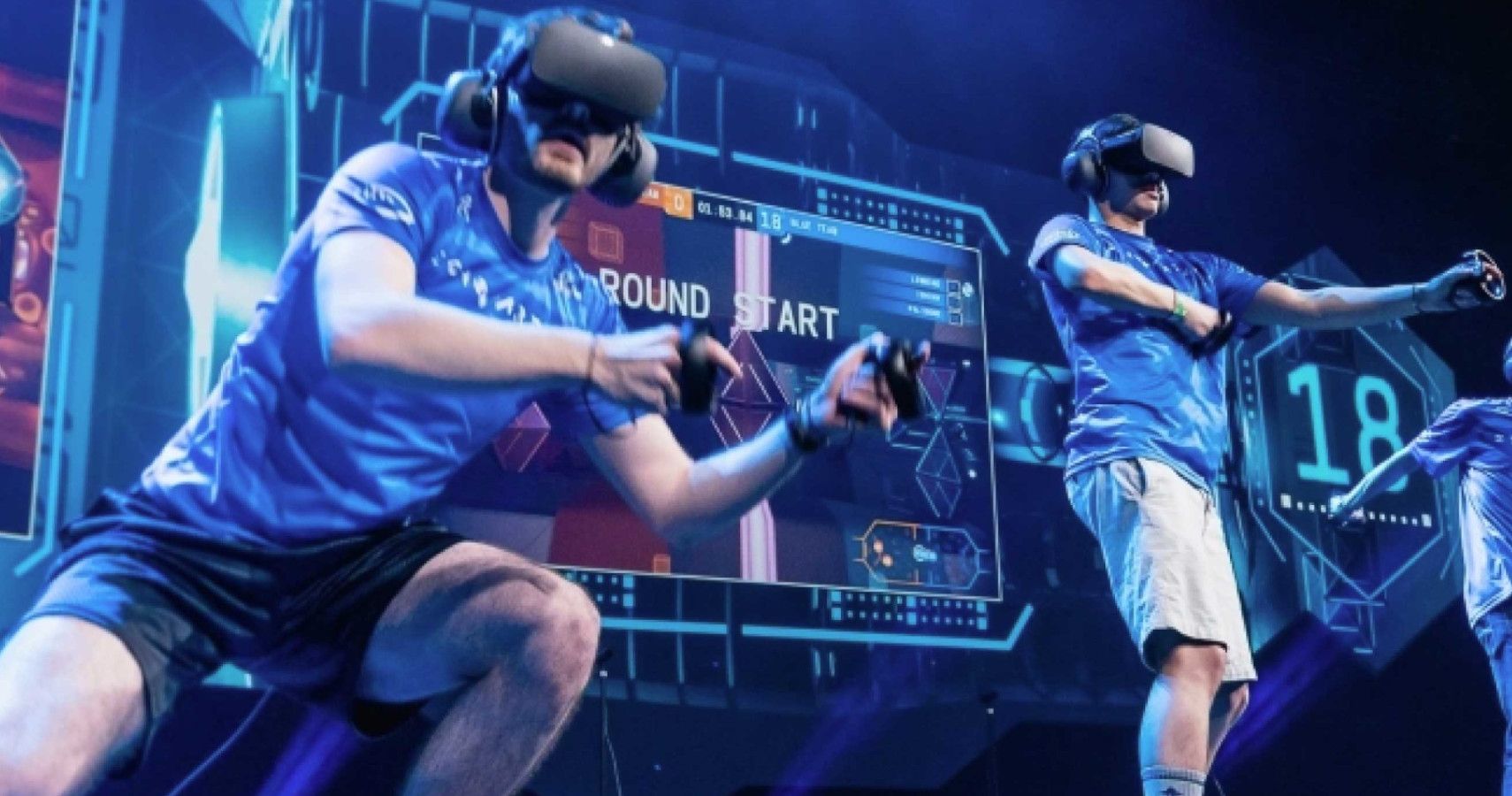The image captures an intense moment of a virtual reality gaming competition featuring two men on a stage. Both players are immersed in the game, wearing blue t-shirts and virtual reality headsets that cover their eyes and ears. They each hold controllers in both hands, with one man dressed in black pants and the other in khaki or cargo shorts. The man on the right appears to be crouching, while his opponent stands more upright. Behind them, a large screen displays the words "Round Start" in white font, illuminating the otherwise dark background. To the right, a sign reads "18." The scene is further enhanced by a spectrum of colors including blue, black, white, gray, orange, yellow, tan, brown, and dark cranberry red. A partially visible third person stands to the far right of the frame, adding to the competitive atmosphere. Though the lighting suggests a well-illuminated stage, the overall feel is more casual than professional, and it is unclear whether an audience is present.